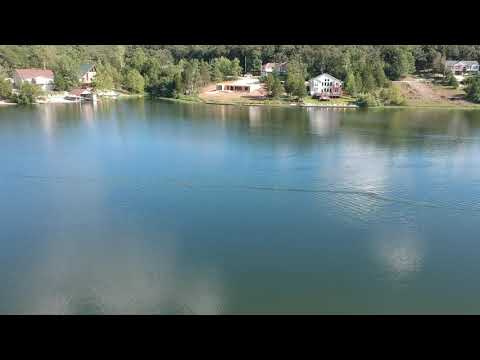The image captures a serene lakeside scene dominated by a large expanse of calm, clear water that reflects sunlight, making the surface appear off-blue. Approximately 85% of the image is composed of the tranquil lake, which showcases subtle ripples particularly at the center. In the background, nestled amidst dense greenery of trees and grass, are several vacation homes. These homes, about four or five in number, are scattered across the top part of the image, with their roofs mostly brown, except for one on the left with a greenish-blue hue. This particular house also features a dock extending into the lake. The homes appear to separate the forested area from the lake, creating a picturesque border. The entire scene, devoid of any human presence, exudes tranquility and the untouched beauty of nature on what appears to be a beautiful day.